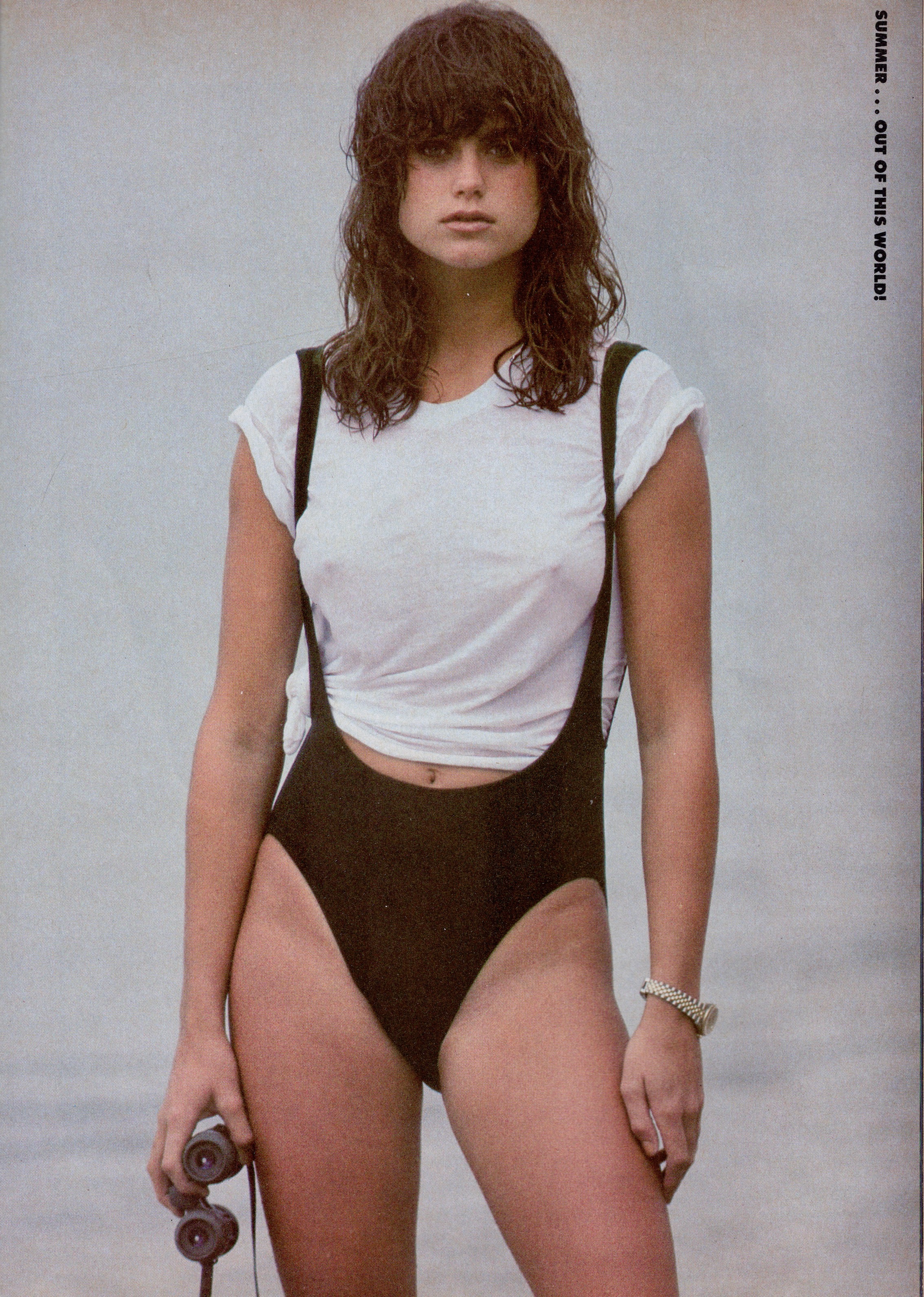The professionally-shot image features a model in a stylish, possibly retro, outfit standing against a greyish-white backdrop. The model, of shoulder-length brown hair and bangs, is staring intently at the camera showcasing a confident, composed demeanor. She wears a white see-through short-sleeve t-shirt over a black unitard that reveals her navel. The unitard includes suspenders that add a fashionable edge to her attire. A touch of sophistication is added with a gold watch on her left wrist. In her right hand, she holds black binoculars, subtly contributing to the ambiance of curiosity and exploration. The muted color palette of black, white, brown, grey, peach, pink, and a hint of gold enhances the modern yet timeless quality of the photograph. There is tiny, unreadable text on one side of the image, and another section of black vertical text in the top right corner that reads, "Summer, out of this world," suggesting a seasonal or thematic promotional message, possibly hinting at an advertisement from the 80s or 90s. The entire scene, void of any additional people or objects, places the model and her ensemble prominently at center stage.